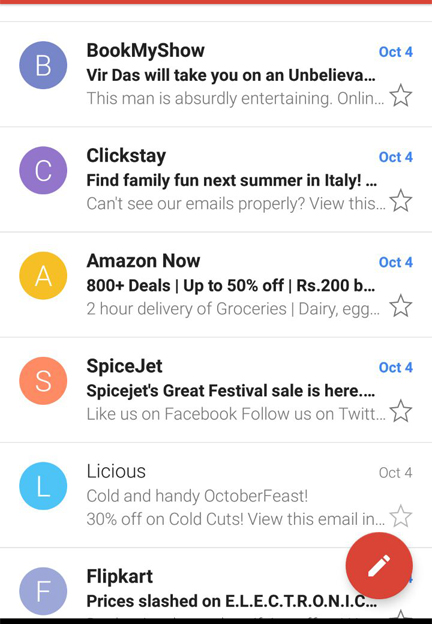In this screenshot of a Gmail account taken on October 4th, several emails are visible in the inbox, though none are fully opened. Here is a detailed description of each email seen in the list:

1. **BookMyShow:** The subject line hints at an event featuring Vir Das, with a partial preview stating, "Vir Das will take you on an unbelievable…,” but the rest of the message is truncated and unreadable.

2. **ClickStay:** This email seems to be promotional, inviting the user to "find family fun next summer in Italy." It also briefly mentions an issue about viewing emails properly with the text, "can’t see our emails properly, view this…," where the message gets cut off.

3. **Amazon Now:** This promotional email announces a sale with "800 plus deals, up to 50% off RS.200B." Another promotional line suggests a fast service, "two-hour delivery of groceries, dairy, egg…," but it is again cut off.

4. **SpiceJet:** This email promotes a sale event titled "SpiceJet's Great Festival Sale is here." It encourages social media engagement with lines like "Like us on Facebook, follow us on Twitter…," which is not fully visible.

5. **Licious:** Advertising an "October Feast," this message promotes a 30% discount on cold cuts, with the preview stating, "Cold and handy October feast, 30% off on cold cuts. View this email in…," before being cut off.

6. **Flipkart:** This email from Flipkart focuses on a sale, indicating that "prices slashed on electronic…," which leads users to believe it's a major sale on electronics but doesn't provide the full details due to truncation.

At the bottom right corner of the screen, the Gmail app's compose button is visible, represented by a red circle with a white pencil icon, enabling the user to create a new email.